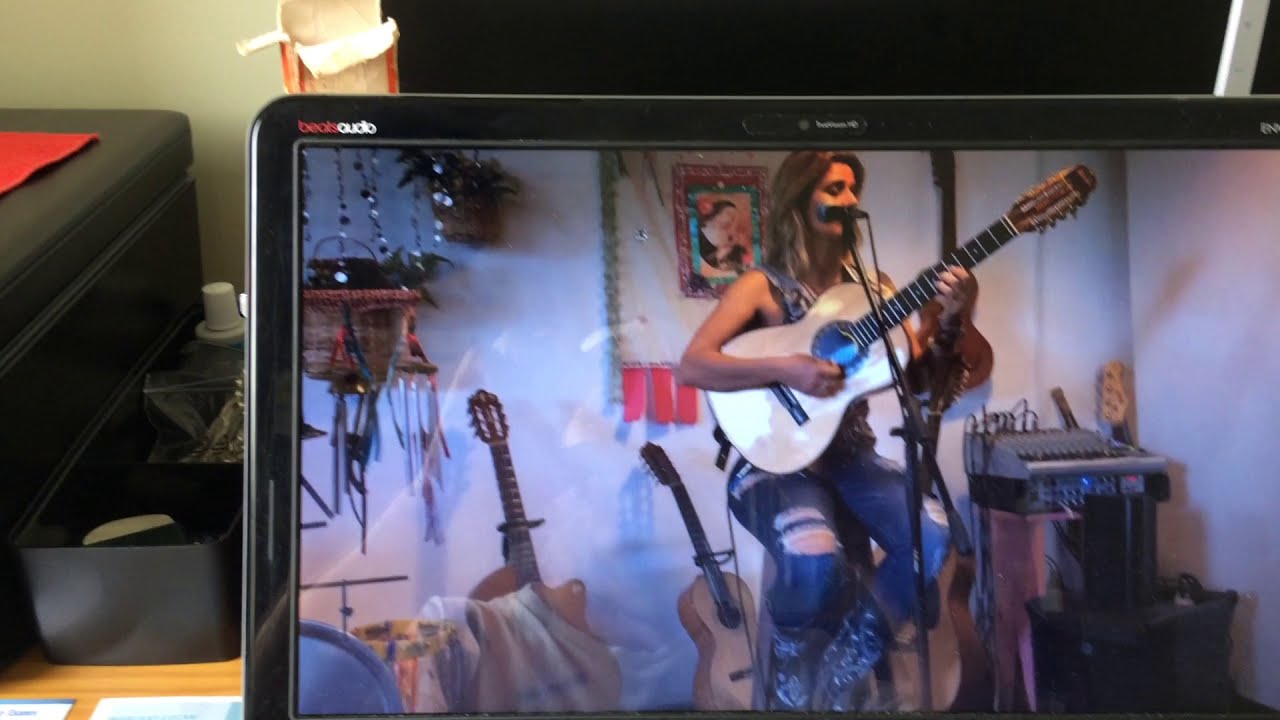The image depicts a digital screen, likely a laptop or touch screen tablet, displaying a close-up of a woman playing an acoustic guitar. She is seated on a stool in a small stage-like area, possibly a bar, wearing boots, ripped blue jeans, and a sleeveless top. Her long brown hair, streaked with blonde, falls to her shoulders. A microphone stand is positioned near her mouth, and she strums a brown guitar with the fretboard angled towards the upper right. Behind her, a white wall adorned with various decorative items and a potted plant hanging from the ceiling is visible. Additional guitars and a keyboard are also in the background, contributing to the musical atmosphere. The digital screen shows the word "beats audio" in the top left corner, with "beats" in red and "audio" in white in lowercase letters. Surrounding the screen on the desktop are miscellaneous items, including the edge of a black container, a black tray with paraphernalia, and a bin containing a plastic bag and a small bottle with a white cap.